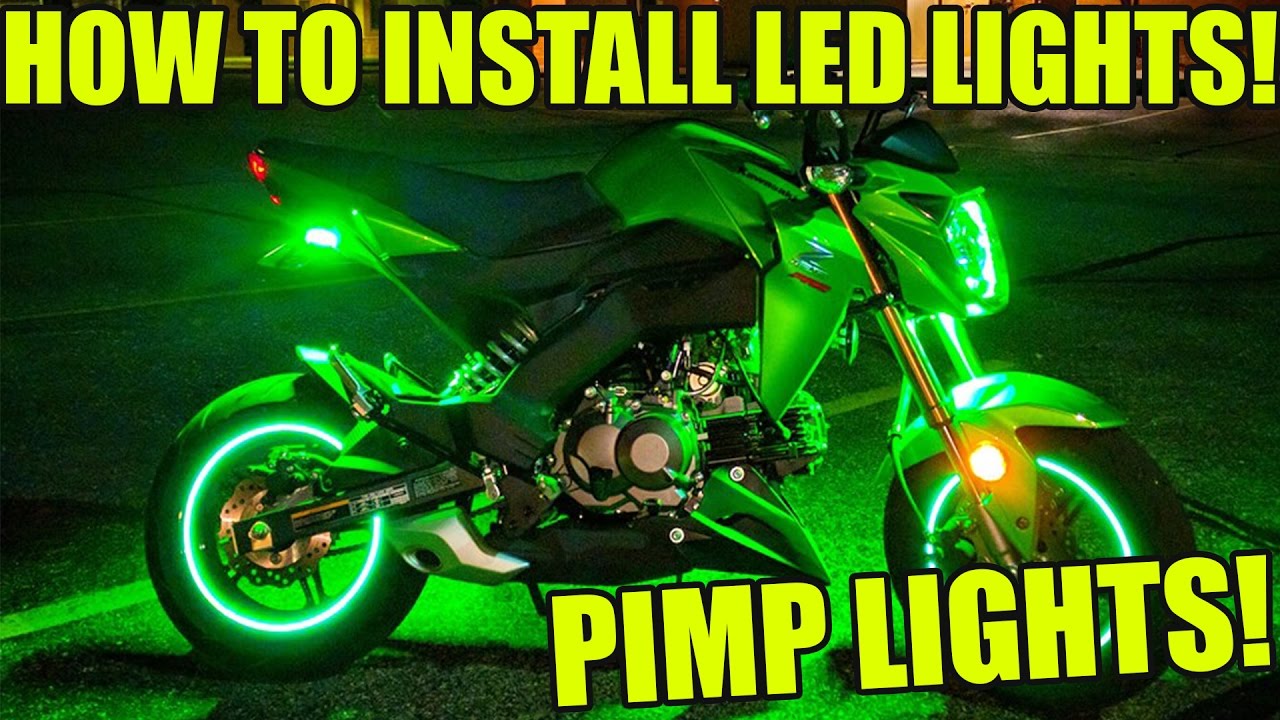The image features a modern Honda Grom or similar small scooter-like motorcycle taken at night in a parking lot. The motorcycle is primarily gray with silver accents on the forks, engine, wheels, and exhaust. LED lights are installed in various locations: beneath the front and rear fenders and around the rims of both wheels, casting a green glow that gives the motorcycle a futuristic appearance. The bike is parked with its kickstand activated, showing no rider in sight. Text overlaid on the image is large, bold, and capitalized with a white font, reading "HOW TO INSTALL LED LIGHTS!" at the top and "PIMP LIGHTS!" in the bottom right corner.